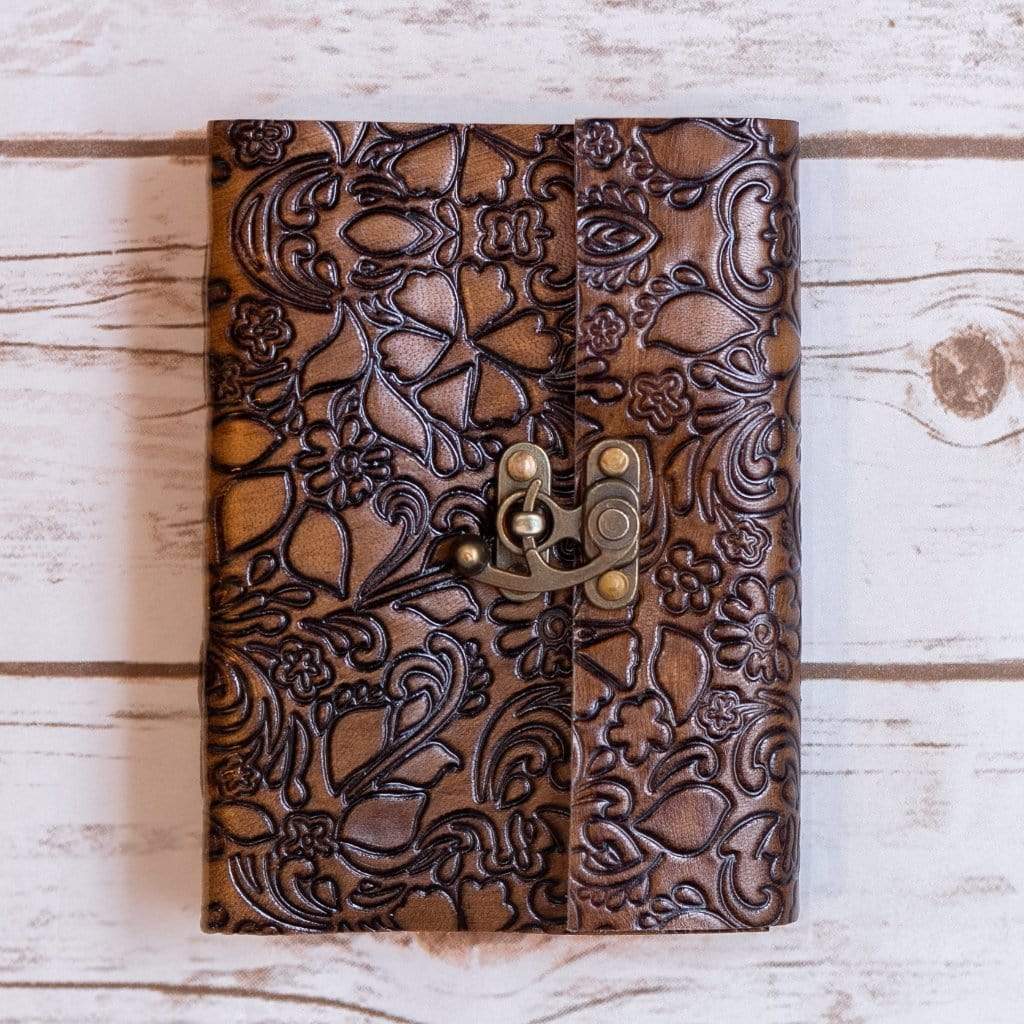The photograph captures a detailed, close-up view of a strapless leather clutch, showcasing a rich brown color accentuated by dark brown to black floral engravings across its rectangular surface. The clutch is meticulously placed on a flat surface designed to resemble white plank wood with dark brown grain lines, although the seamless connections between the 'planks' reveal it is a printed pattern. The clutch itself is oriented with its longer sides horizontally aligned, and its clasp mechanism, located at the center, features a bronze, oval-shaped design with metal hooks and studs. The flap closes by rotating a small hook into a corresponding ring. The image exudes clarity and brightness, emphasizing the tactile detail of the leather material and intricate engravings, set against the light-colored, faux wooden backdrop.